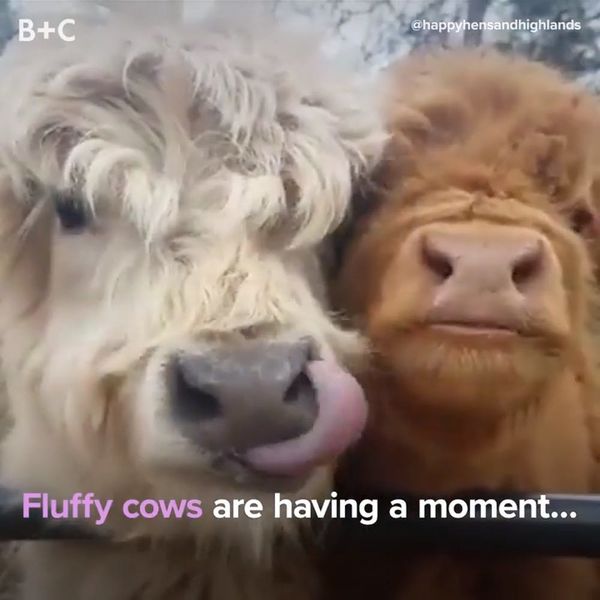This image showcases a detailed close-up of two fluffy cows, filling most of the frame with their faces. The cow on the left features long, white, and fuzzy hair with one dark eye visible beneath the hair. Its gray nose is being tickled by its tongue, which is curled upwards into its nostril. The cow on the right, slightly out of focus, is a rich brown color and similarly fluffy, with its nostrils and mouth prominently displayed. Both cows have such dense fur that their eyes are partly obscured. The background consists of bare tree limbs and trunks, suggesting a non-green, possibly wintry setting. Text overlays occupy the corners of the image: "B+C" in white text on the top left, and an Instagram handle "@happyhensandhighlands" on the top right. Across the bottom, the caption reads, "Fluffy cows are having a moment..." with "Fluffy cows" in pink text and the rest in white.